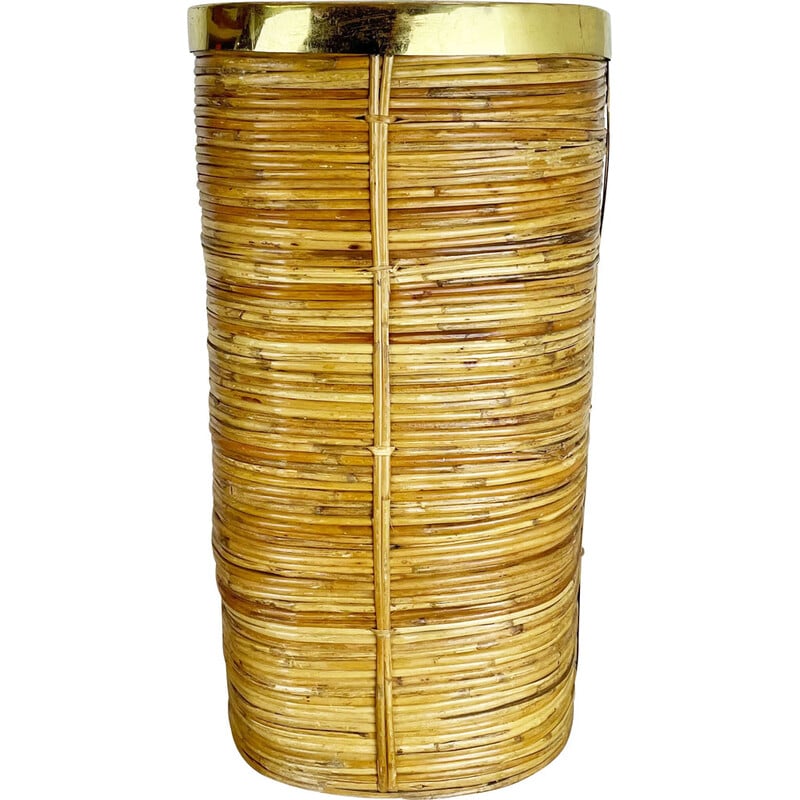A beautifully crafted, tall and narrow container made from interwoven strips of rattan in varying shades from dark streaks to pale hues, showcasing a natural gradient. The rattan strips are meticulously wound in a circular pattern and secured with vertical double pieces of rattan, giving the container both elegance and sturdy structure. This rustic yet refined piece is topped with a shiny, brass-colored lid, adding a touch of sophistication to its earthy aesthetic. Ideal for storing food or dry goods, this container blends functionality with charming craftsmanship.